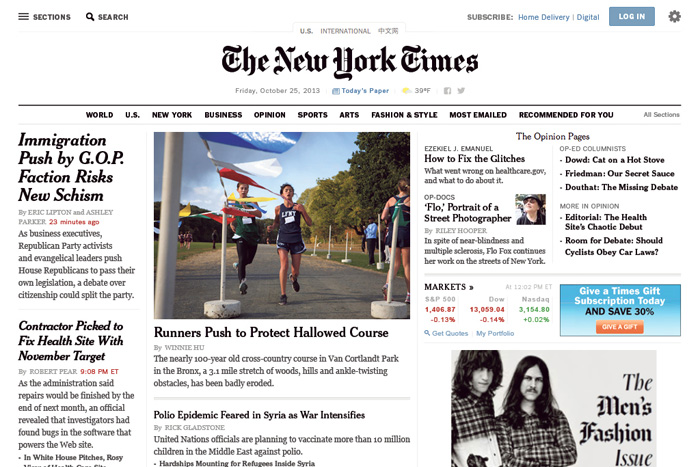The webpage displays a structured layout with distinct sections:

- On the top right, there are three horizontal lines labeled "Sections," followed by a magnifying glass icon for "Search."
- On the left, there are options for "Subscribe" and a blue "Home Delivery" link.
- A blue box for "Log In" is adjacent to a gear icon, with smaller, unreadable text in black beneath it.
- The header prominently displays "The New York Times" along with the current date. There is a blue link with a yellow spot and adjoining text, alongside two gray icons.
- A black line separates the header from a navigation bar that reads: "World," "U.S.," "New York," "Business," "Opinion," "Sports," "Arts," "Fashion & Style," followed by partially readable sections including "Recommended For You" and "All Sections."
- On the left side, a headline reads "Immigration Push by GOP Faction Risks New Schism," with additional text beneath it.
- Below, another headline states, "Contractor Picked to Fix Health Site with November Target," followed by more text.
- On the right side, an image depicts people running, captioned "Runners Pushed to Protect Hallowed Course," with further text that is too small to read.
- The "Opinion Pages" section is mentioned with accompanying unreadable text in black and a small square image of a person’s face.
- A "Markets" section is underlined by a gray line, featuring unreadable gray numbers, followed by red numbers underneath, with blue numbers adjacent and green numbers on the far right.
- A darker blue rectangle at the far right promotes a "Give a Times Gift Subscription Today and Save 30%," followed by an orange rectangle with unreadable text.
- At the bottom, a picture of two men with long hair and checkered shirts touts "The Men's Fashion Issue."

This detailed layout captures the essence and intricacies of the New York Times webpage.